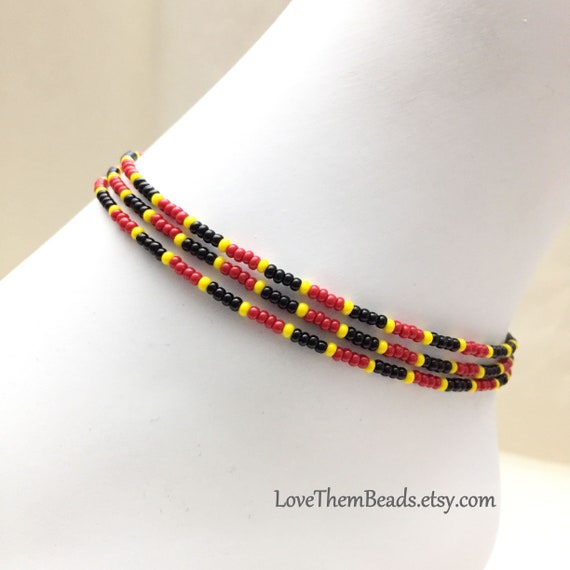This image displays a fashion accessory product, specifically an anklet, elegantly showcased on a mannequin leg. The anklet features a striking design consisting of three distinct rows, each meticulously crafted with black, yellow, and red beads. The beads are systematically arranged in a repeating pattern of black, yellow, red, black, yellow, red, ensuring a harmonious and balanced appearance across all rows.

The white surface under the mannequin leg distinctly contrasts with the vibrant colors of the beads, highlighting the anklet's intricate design. The background features a beige wall, providing a neutral and understated backdrop that allows the anklet to be the focal point of the image. Additionally, in the bottom right corner, the text "lovethembeads.hetzy.com" is prominently displayed in black font, indicating the source or brand associated with this stylish accessory.